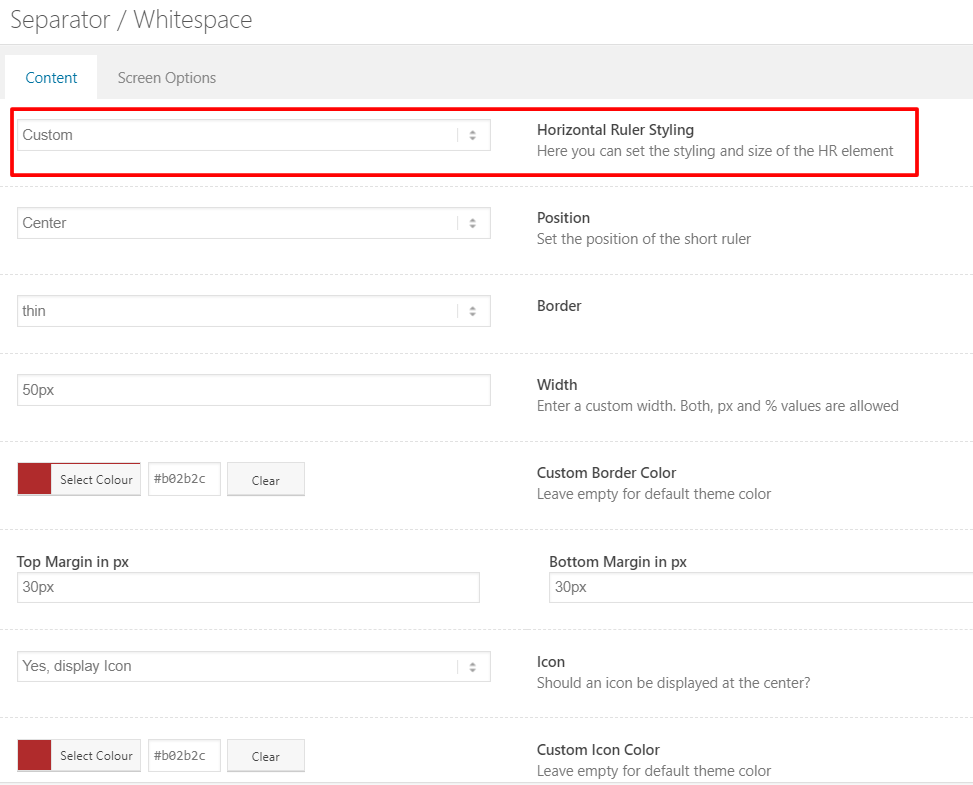The image is a screenshot from an image editing application, featuring a predominantly white background. The top left corner displays gray text that reads "separator / whitespace." Directly below, there is a horizontal gray bar that represents the menu options of the application. The menu shows various options with "Content" highlighted in blue text within a white box, indicating that the "Content" tab or section is currently active. Next to "Content," in light gray text, is "Screen Options."

Central to the image and extending to the bottom, there are various options for editing a photo. These options include settings like "Horizontal Ruler Styling," "Border," "Custom Border Color," "Margin," among others. The topmost option, "Horizontal Ruler Styling," is enclosed in a red box, highlighting it as the selected option. This section allows users to customize the styling and size of the horizontal ruler (HR) element. To the left of this option is a drop-down box featuring the word "custom," implying that the user can personalize the horizontal ruler styling.

The other options are presented in standard black or gray text against a white background, offering various image editing functionalities. The overall design suggests a user-friendly interface aimed at facilitating detailed photo edits.